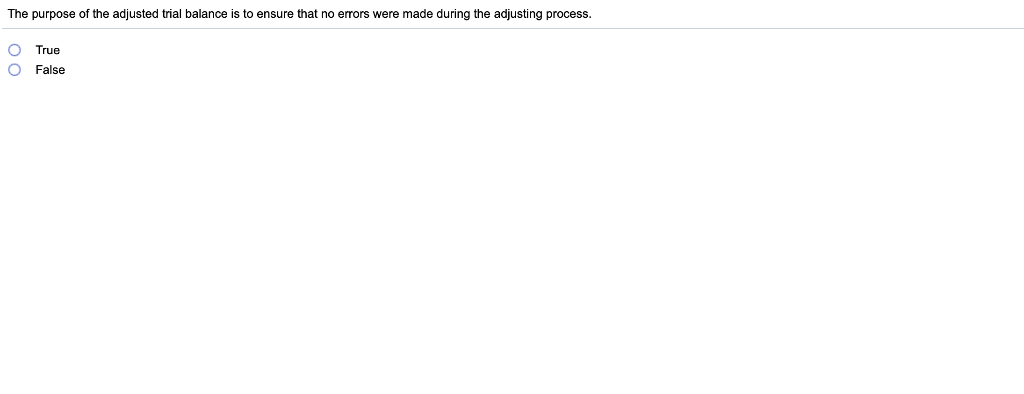The image features a completely white background with no additional details or elements. At the center of the image, there is informative text stating, "The purpose of the adjusted trial balance is to ensure that no errors were made during the adjusting process." Below this statement, there are two options available: "True" and "False," indicating a multiple-choice format. It is noted that neither of these options has been selected. The text is repeated verbatim further down the page. The stark white background creates a minimalistic and clean presentation, emphasizing the textual content and the absence of any other graphical elements.